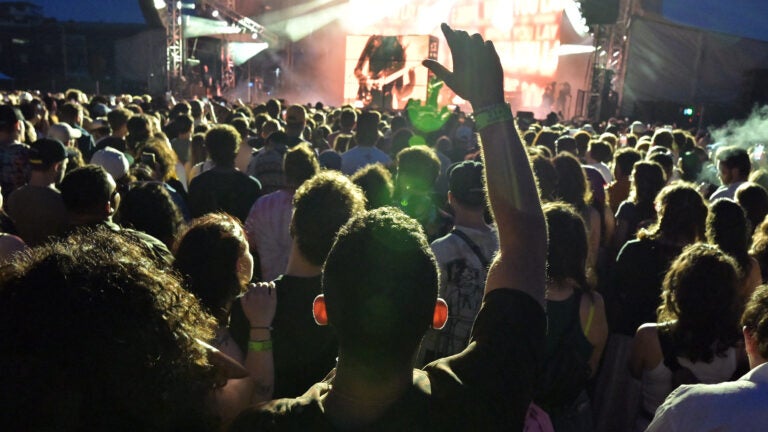This detailed photograph captures the energized atmosphere of an outdoor music festival at night. Taken from within the audience toward the back, the image is filled with the backs and heads of numerous attendees, creating a sea of dark silhouettes. Central to the scene is a man directly in front of the camera, his right arm raised high, the light from the stage illuminating his wristwatch and giving his ears an almost glowing appearance. Up ahead on the brightly lit stage, a large screen prominently displays a musician passionately playing an electric guitar, clad in dark clothes. Flanked by unlit white canopies, the stage stands out against the dark night sky, with dynamic lighting adding to the vibrant ambience of the concert.